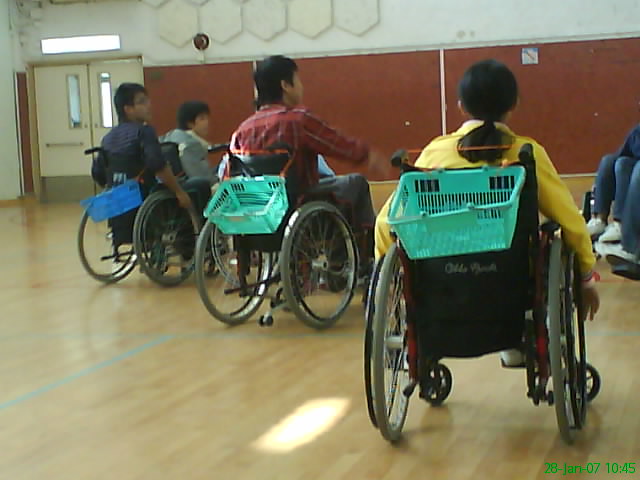The photo captures a group of six individuals, primarily of Asian descent, seated in wheelchairs arranged in a circular formation on the wooden floor of a gymnasium, likely a school setting. The gym features a distinctive wall with a red lower half and a white upper half, accompanied by beige double doors providing an exit. Each wheelchair has a plastic shopping basket strapped to its back—two with light blue baskets, one with a dark blue basket, and some with indeterminate colors. The wheelchair closest to the viewer boasts a partially red frame. The individuals are arrayed facing each other, possibly for an activity or discussion. The woman closest to the viewer is dressed in a yellow long-sleeved top and has her long hair tied back. To her left, a man wears a red checkered shirt and gray jeans, and further left, another individual sports a long-sleeved blue shirt and glasses. Some of the other individuals are indistinct, but those visible are clad in white sneakers and blue jeans. The timestamp at the bottom of the image, though hard to read, indicates the photo was taken on January 28, 2007, at 10:45 AM.